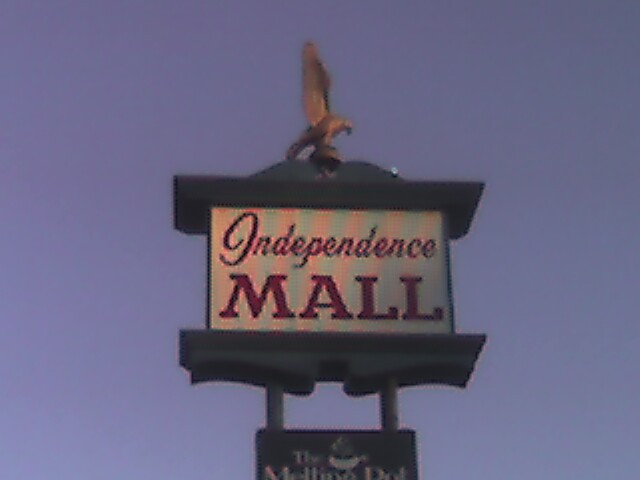This image features a large, imposing sign reaching high into the sky with no treetops or other objects visible. The top portion of the sign boasts the name "Independence Mall," with the word "Independence" elegantly written in red script, while "Mall" is in bold, red block lettering, all set against a light-colored background. Crowning the sign is a golden eagle with its wings majestically spread wide, perched atop a scalloped wooden platform. The sign is supported by two cylindrical poles matching the sign's dark blue-black color scheme, and beneath the primary signage is an additional panel that reads "The Melting Pot," which is a restaurant. This lower section features an illustration of a pot, reminiscent of a kettle, symbolizing the restaurant's theme.